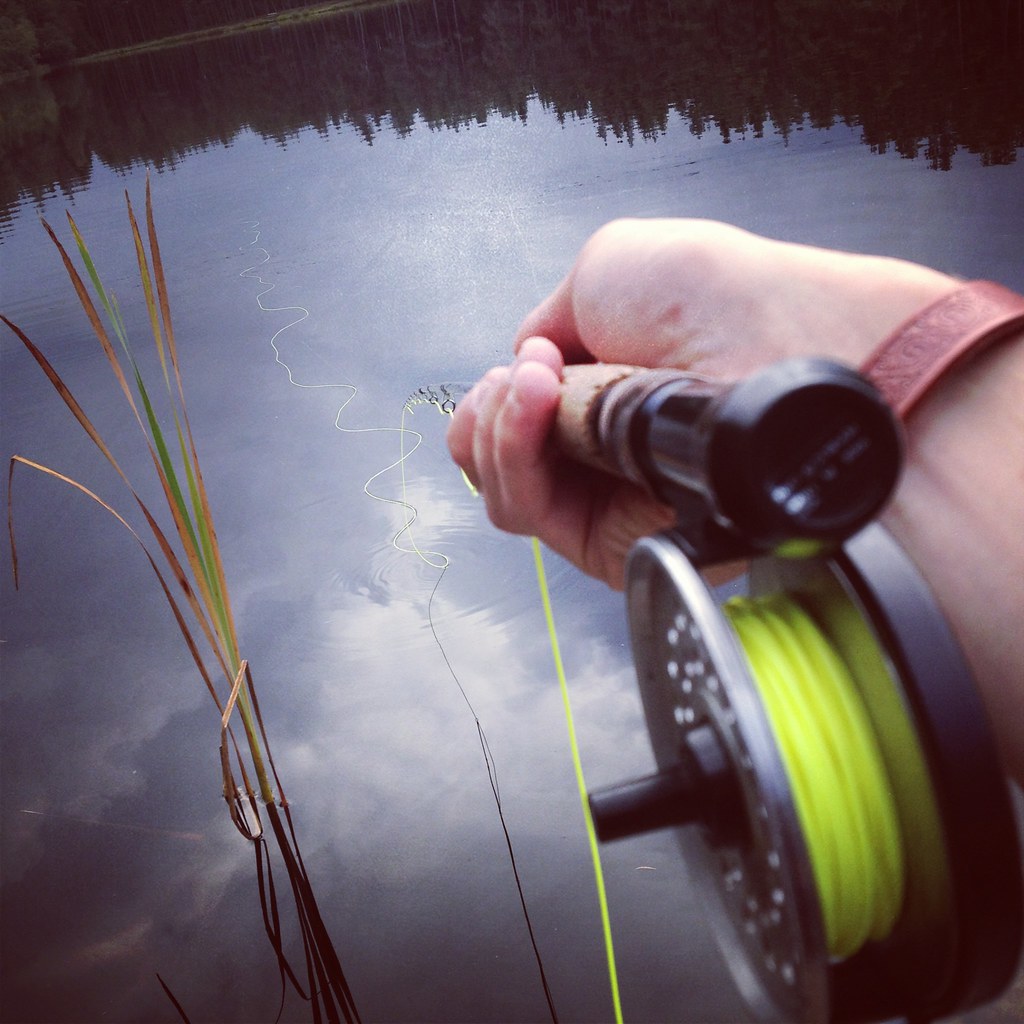A close-up capture of an angler's right hand holding a fishing reel dominates the frame. The hand is adorned with a red band, possibly a wristwatch partially obscured. The fishing line, a distinctive yellow hue, is cast into the calm body of water below. The water's surface subtly mirrors the silhouette of trees along the upper edge of the image, adding a natural border. On the left side of the angler, tall grass sways gently, framing the serene fishing scene. The photograph meticulously details the intimate connection between the fisher and their craft, against a backdrop of tranquil waters and reflected greenery.